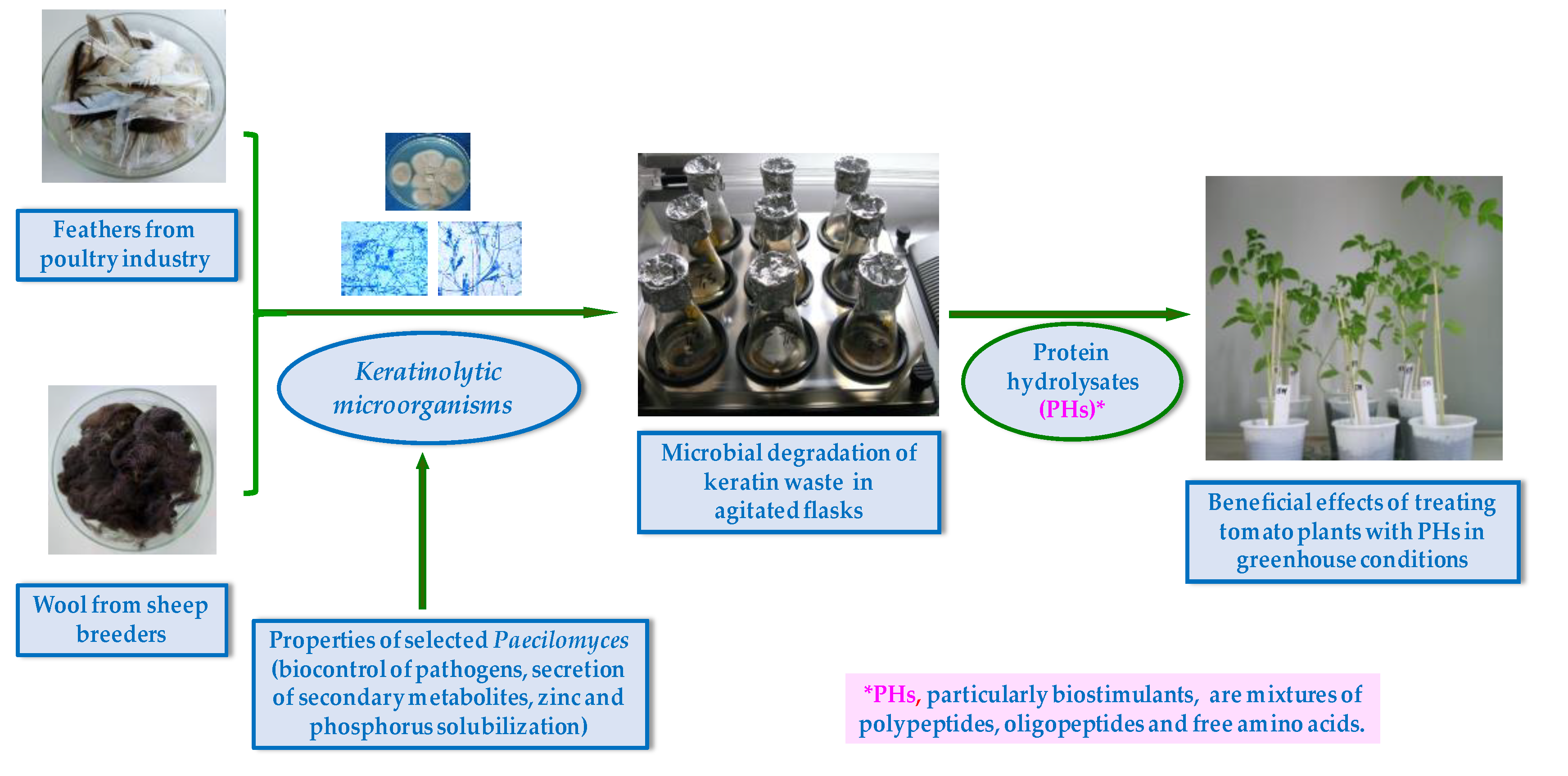This diagram, resembling a detailed agricultural or biochemical flowchart, outlines the process from keratin waste materials to beneficial agricultural applications. Starting at the left, it features a picture of feathers from the poultry industry and black wool from sheep breeders, each housed in a separate container, symbolizing the raw materials. Arrows guide the viewer to the next stage, highlighting the role of carotenolytic microorganisms in the biocontrol of pathogens, the secretion of secondary metabolites, and the solubilization of zinc and phosphorus. Following this, the process shows microbial degradation of keratin waste in agitated flasks, represented by a trio of flasks on a shaking machine. The final phase leads to the creation of protein hydrolysates (PHS), noted for their beneficial effects on tomato plants. This is visually depicted with the healthy growth of tomato plants treated with PHS in greenhouse conditions, capturing the full journey from animal-derived waste to agricultural productivity.